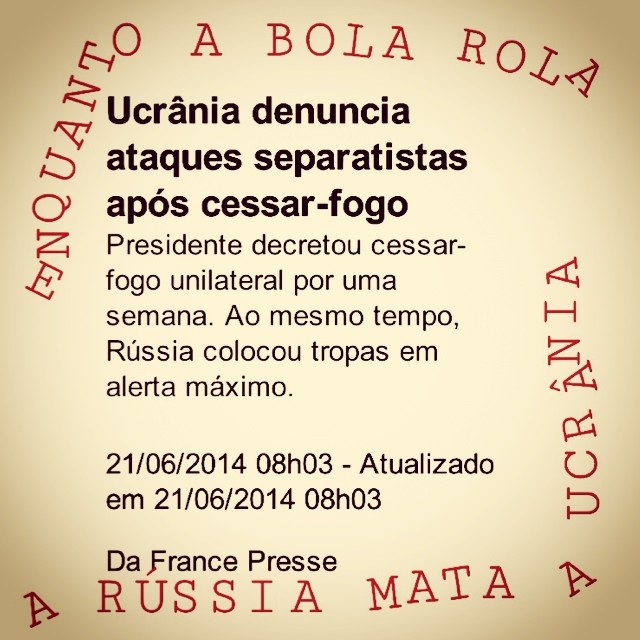The image displays a flyer with a yellowish-white background and text in both red and black. In the upper left corner, text in red all-caps reads "EM QUANTO A BOLA ROLA," running vertically before turning horizontal across the top. The lower part of the flyer also features red, slightly crooked text stating "A RÚSSIA MATA A," and running up the right-hand side, it spells out "UCRÂNIA." The central message is in black text, starting with "UCRÂNIA DENUNCIA," followed by several lines in the same dark black font, which appear to be in either Spanish or Portuguese. Key phrases include "PRESIDENTE," "RÚSSIA," "MÁXIMO," and "TROPAS." Notable terms like "ALERTA MÁXIMA" suggest it may be an urgent message or alert. Numbers and the name "DA FRANCE PRESSE" are listed at the bottom, indicating a potential news source. The use of bold black text at the top emphasizes the importance of the main message.